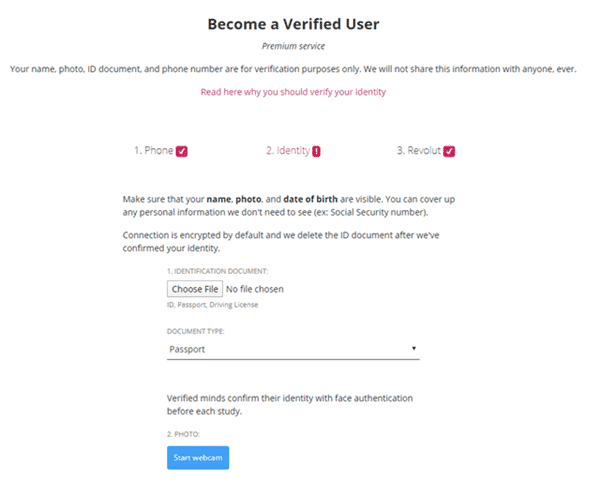The web page for becoming a verified user is prominently displayed with a clean and clear design. Dominating the page are the words "Become a Verified User" written in big, bold, black letters. Below this, the term "Premium Service" is indicated, suggesting that this verification offers enhanced features or benefits.

In smaller print, a reassuring message reads: "Your name, photo, ID document, and phone number are for verification purposes only. We will not share this information with anyone ever." This emphasizes the importance of user privacy and data security.

In striking red print, there's a link labeled "Read here why you should verify your identity," inviting users to understand the benefits and importance of the verification process.

The layout on the white background is organized with a clear step-by-step guide:

1. **Phone**: Accompanied by a red square with a check mark.
2. **Identify**: Clearly written in red and highlighted as step number two with a corresponding red number.
3. **Revolut**: Marked as step number three, also checked off with a red box.

Further instructions clarify that users need to ensure their **name, photo, and date of birth**—all bolded for emphasis—are visible. They are advised that any non-essential personal information, like a social security number, can be covered up.

Additionally, the page assures that the connection is encrypted by default, and it emphasizes that ID numbers are deleted after confirmation to maintain security.

For the identification document, there are options to choose or upload a file, with examples provided (e.g., passport, driving license). Users can select the document type from a dropdown menu.

There's also a section stating: "Verified" indicating that verification of identity will involve authentication before each study. Finally, there's an option to use a webcam to start the photo verification process.

Overall, the page is meticulously designed to guide users through the verification process while emphasizing security and privacy.